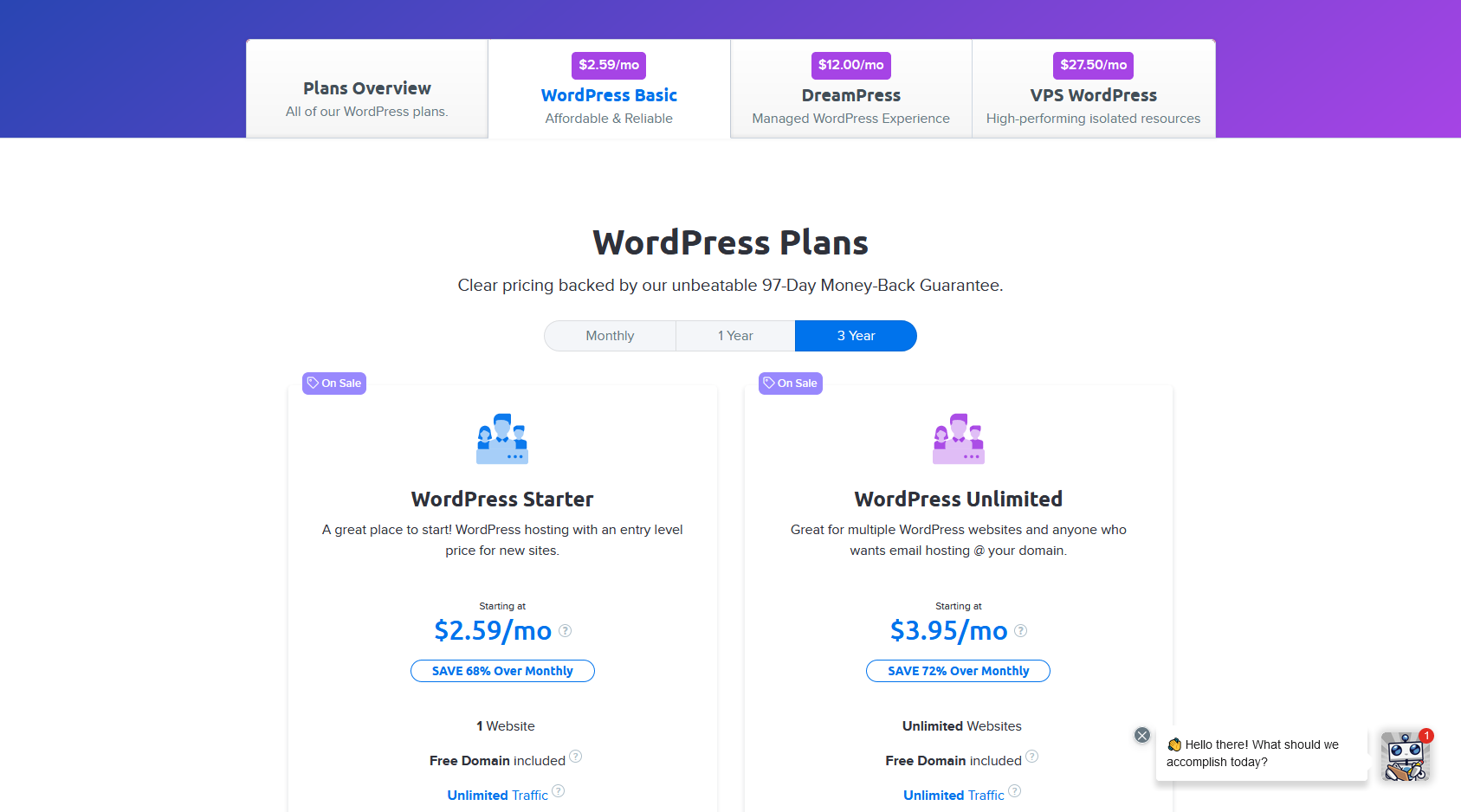This screenshot provides an overview of various WordPress hosting plans, clearly showcasing different payment options. 

The top of the image prominently features a "Plans Overview" title. Directly below, the section breaks down three primary plans: "WordPress Basic" for $2.59 per month, "DreamPress" for $12 per month, and "VPS WordPress" for $27.50 per month. 

In the middle of the image, a banner states "WordPress Plans: Clear pricing backed by our unbeatable 97-day money-back guarantee," accentuating customer assurance. 

Further down, there are three tabs that indicate different subscription durations: "Monthly," "One-Year," and "Three-Year," with the "Three-Year" tab highlighted in blue.

On the left side, there is detailed information about the "WordPress Starter" plan, described as a great entry-level hosting option for new sites, priced at $2.59 per month, promising a 65% saving over the monthly plan.

On the right, the "WordPress Unlimited" plan is highlighted, designed for users with multiple websites, available at $3.95 per month.

This comprehensive image effectively delineates WordPress hosting options, targeted at both beginners and advanced users with multiple sites.